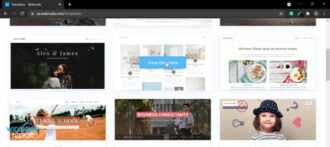This image appears to be a detailed screenshot of a webpage viewed from a computer or laptop. The image is narrow, approximately two inches long, with a wider bottom section. At the very top, there is a gray tab indicating an open browser tab, situated next to a black bar that spans across the screen. Below this is a gray bar positioned at the upper left corner, containing a blue box with white text inside. Adjacent to this blue box are typical webpage icons.

Continuing down, there's another gray box featuring three icons on the left, followed by a search bar with white text inside. On the right of this search bar, there are five more icons, starting with a green circle.

Beneath this section, the layout features several boxes. The top row shows the bottom portions of three boxes: one gray, one white, and another gray from left to right. Directly below this, a black-background box contains two figures. Right next to it, a white box holds a blue bar with more white text at its center. Following this, another white box displays two side-by-side images of fancy platters, reminiscent of Instagram photos.

Further down, an orange field box presents a figure standing in front of it. This field prominently displays an outdoor image of a man wearing a white button-up shirt, overlaid with a red box containing white text. 

In the bottom right corner, next to the man, there is a photograph of a young toddler with brown hair, wearing a black hat and a white-and-blue striped shirt.